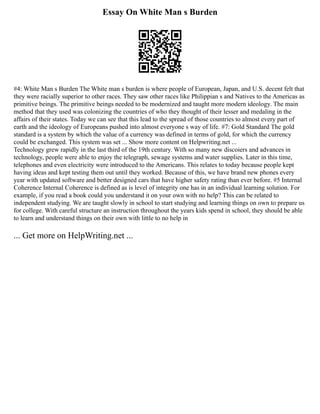The image displays a small, poor-quality photograph of text titled "Essay on White Man's Burden" at the top. Directly below the title, there's a QR code, presumably leading to additional information. The main body of the text is a paragraph discussing the concept of the White Man's Burden, where people of European, Japanese, and U.S. descent believed they were racially superior to others, perceiving races such as Filipinos and Native Americans as primitive beings needing modernization and colonization. The image is entirely in black and white, making the already minuscule and difficult-to-read print even harder to decipher. Separate from the main paragraph, at the bottom, there is a line of text promoting a website, helpwriting.net, which offers resources for overcoming writer's block and improving writing skills.